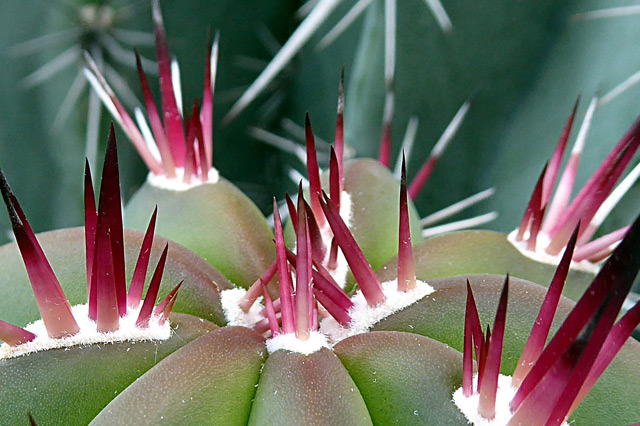This extreme close-up image showcases two cacti, one prominently in the foreground and another in the background. The cactus in the foreground features striking green plant bases with reddish hues that intensify to pink and then dark red near their tips, almost black at the ends. Emerging from a fuzzy white substance at the base, each cluster of spikes displays a gradient, starting light and becoming more vibrant and dark toward the tips. There are multiple clusters, each radiating around eight to ten sharp spikes. 

In contrast, the background cactus, though blurred, reveals a bluish-green color and white spikes that are larger and darker toward their bases. The overall texture of this cactus appears more ridged and lumpier compared to the smoother, rounder foreground cactus. The detailed view captures the intriguing differences in colors and textures, bringing out the vivid purples, reds, greens, and whites of the spikier foreground cactus vividly against the hazier background.